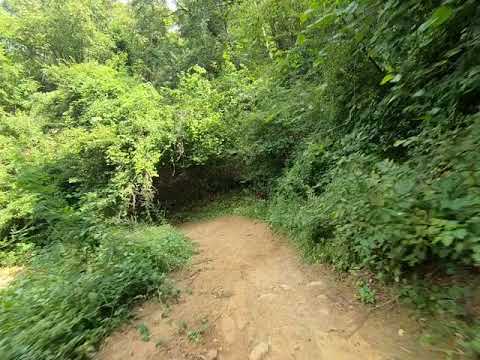The image depicts a serene woodland path during the day. The central focus is a narrow dirt trail, slightly wider than a typical sidewalk, descending down a hill and curving gently to the left, creating the illusion of a natural tunnel formed by the dense vegetation surrounding it. The path is well-trodden and relatively flat, with occasional small rocks scattered across its brown surface.

On either side, as well as above, the trail is flanked by lush greenery, including trees, bushes, and grass, all vibrant and healthy, indicating a well-watered environment. The canopy of trees overhead forms an arch, casting the path into a shadowy, almost tunnel-like atmosphere as it winds into the shaded depths of the forest.

Though the sky is mostly obscured by the thick foliage, faint patches of light peek through the leaves, hinting at a bright, sunlit day outside the dense cover. In the upper center-left of the image, there is a small break in the canopy where the sky is just visible, appearing somewhat white, possibly due to the light filtering through or the presence of clouds.